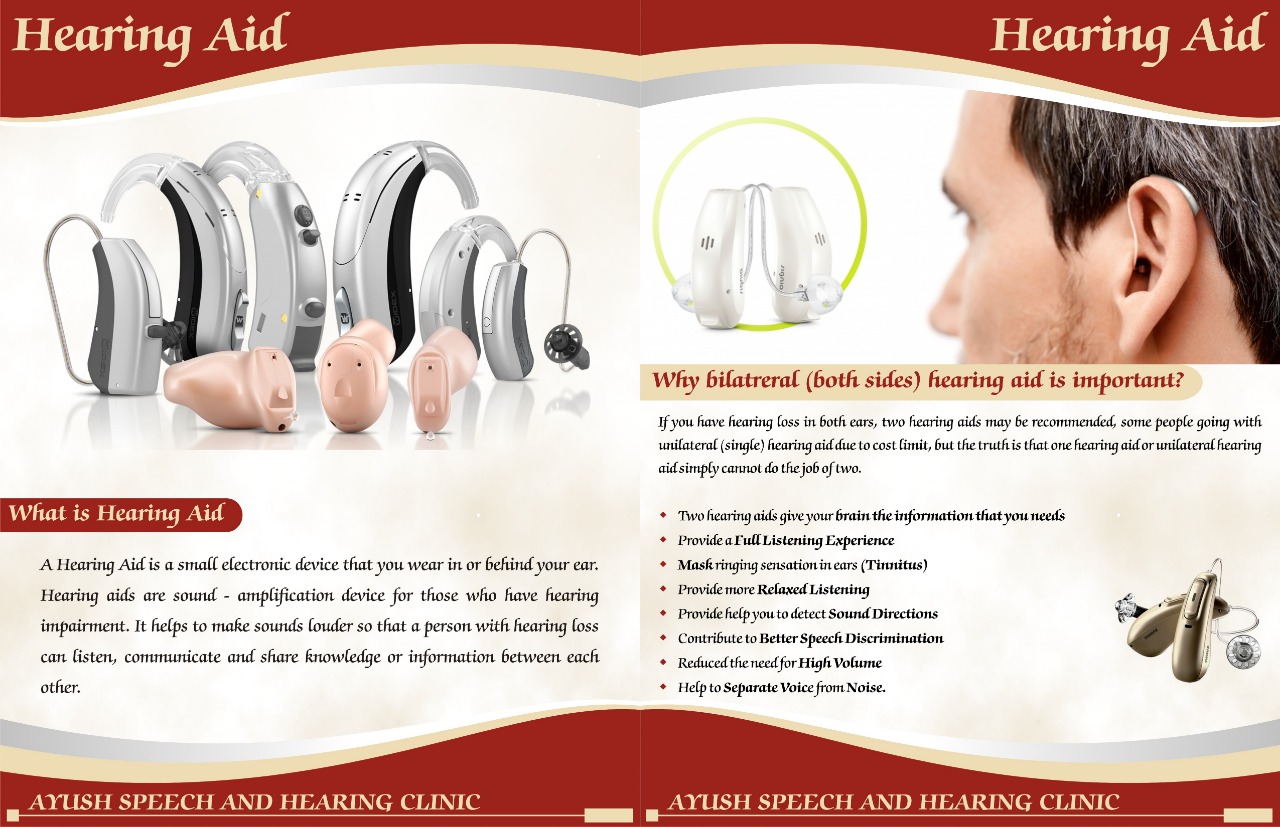The image is an advertisement for hearing aids displayed as a two-page catalogue spread. Both pages feature a repeating swirly red border at the top and bottom. On the left page, prominent text in a beige font reads "Hearing Aid" in the upper left corner. The main focus of this page is a large image displaying various models of hearing aids. The hearing aids include larger silver ones in the background and sleeker, minimalistic models in a metallic pinkish-beige and grey-silver color in the foreground. Beneath these images is a detailed paragraph explaining what a hearing aid is: a small electronic device worn in or behind the ear to amplify sound for those with hearing loss, helping them to communicate better. The bottom of this page prominently features the name "AYUSH Speech and Hearing Clinic."

On the right page, the top right corner also displays the text "Hearing Aid" in the same beige font. This page includes another image showing a man wearing a hearing aid, demonstrating its fit and appearance in the ear. Below this image, a bullet-point list outlines the benefits of using hearing aids, emphasizing their importance and effectiveness in improving hearing and communication. At the bottom of this page, the text "AYUSH Speech and Hearing Clinic" is repeated, reinforcing the brand identity.